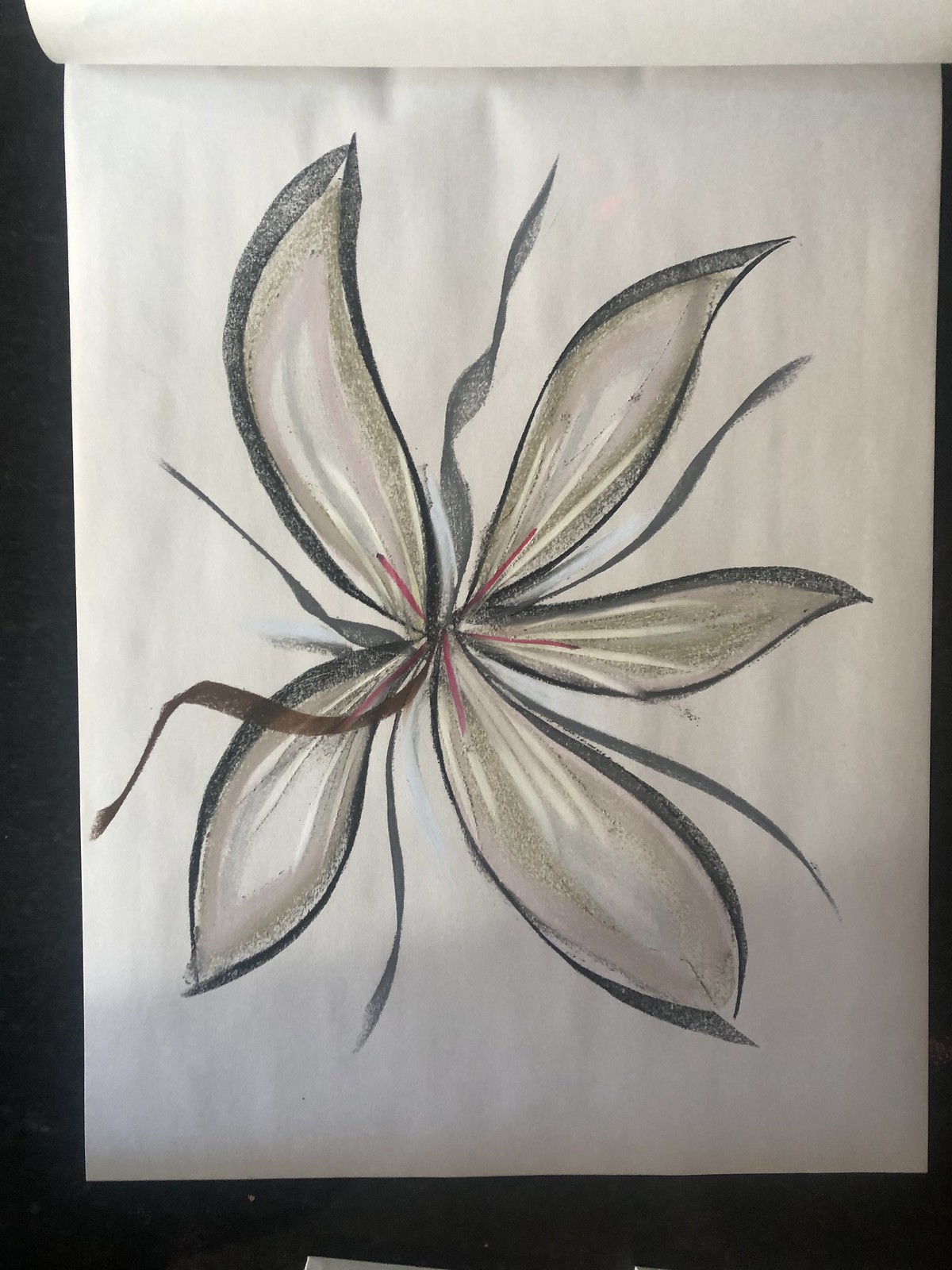This vertically-oriented rectangular photograph captures an intricately drawn flower on a slightly creased and wrinkled piece of white paper. The flower features five elongated petals that are a blend of gray, green, and a subtle pink hue. Radiating from the center, thick, squiggly black lines extend between each petal, adding dynamic texture to the image. Prominent red stamens also emerge from the flower's core, introducing a striking contrast. Additionally, a long, squiggly, flat brown line starts at the center of the flower and gracefully curves down to the bottom left corner of the paper. The vivid illustration is set against a stark, jet-black backdrop, enhancing the visual impact of both the drawing and the paper's textures.